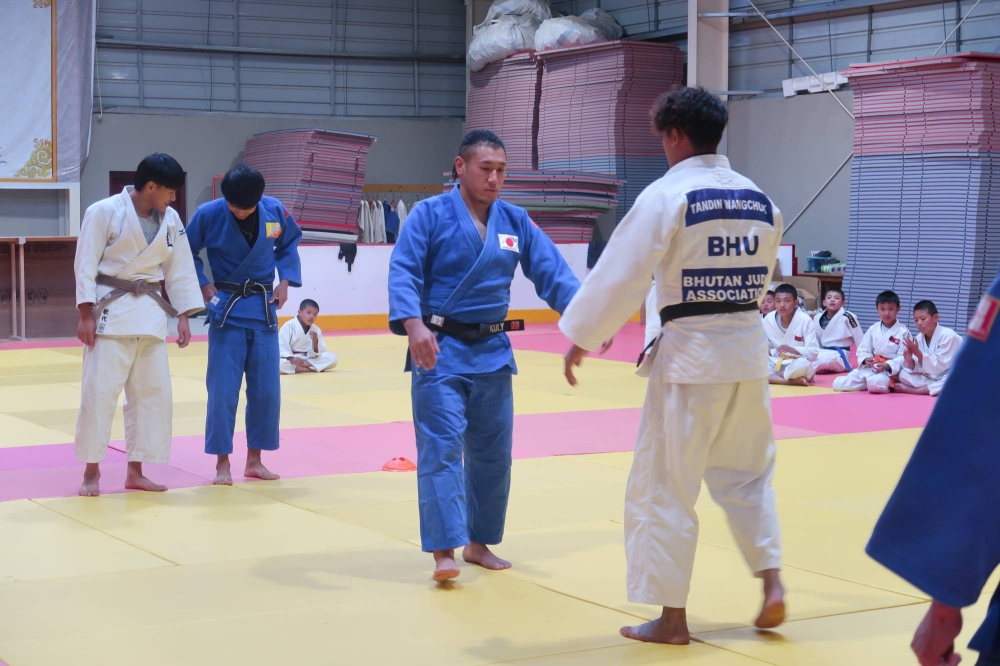The photograph depicts an indoor judo match taking place within a gymnasium-like dojo with high gray walls and a wooden floor covered in yellow and pink mats. Two Asian men are the primary focus; the one on the right is dressed in a white gi with black bars, white lettering, and a "BHU" label on the back, while the man on the left, facing the opponent, wears a light blue gi adorned with a white patch featuring Japan’s flag. Both men have dark black hair, wear black belts, and stand barefoot in a sparring position with their arms slightly outstretched toward each other. Behind them stand two more men; one in a white gi with a tan belt and another in a light blue gi with a black belt, slightly watching the match. Further back, a group of younger students dressed in white gi are seated cross-legged on the floor, attentively observing the ongoing contest. The gymnasium's background features stacks of padded mats, enhancing the dojo’s authentic martial arts atmosphere. The detailed setting and participants suggest a vigorously engaging judo practice session under the Bhutan Judo Association.